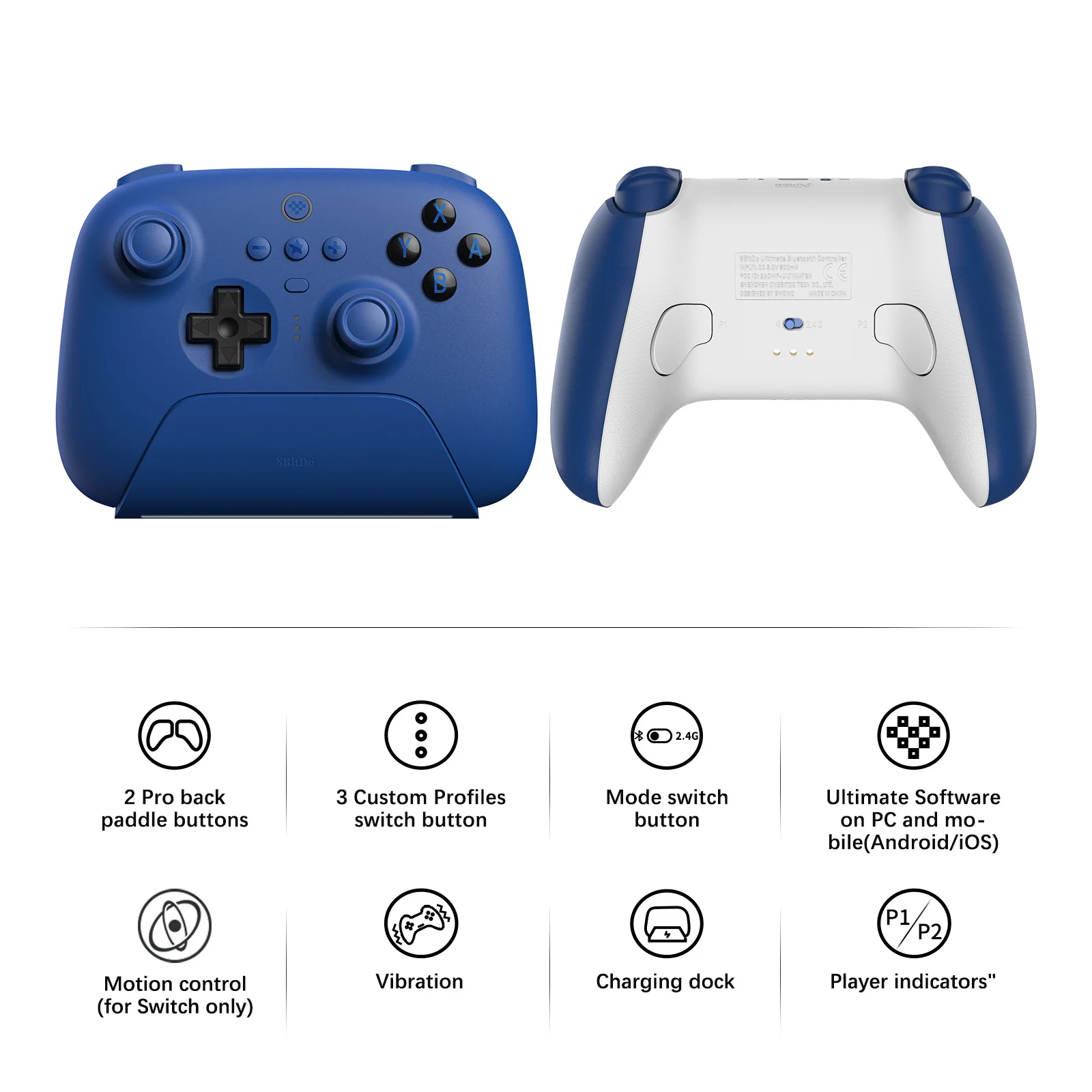The image showcases a sophisticated video game controller in two views, one from the front and the other from the back. The front view highlights the controller's deep blue color with black accents, including black joysticks and a black D-pad. In the center are three additional buttons, and above them is a small, round power button. The controller also features black X, A, Y, and B buttons on the upper right side. The back of the controller has blue sides and a white central portion, contributing to its ergonomic design.

Below the images of the controller are detailed descriptions and icons specifying various features. These features include two ProPack paddle buttons, motion control for Switch only, three custom profile switch buttons, vibration, a mode switch button, compatibility with ultimate software on PC and mobile (Android/iOS), a charging dock, and player indicators. This visually appealing and functional controller is perfectly designed for an immersive gaming experience.